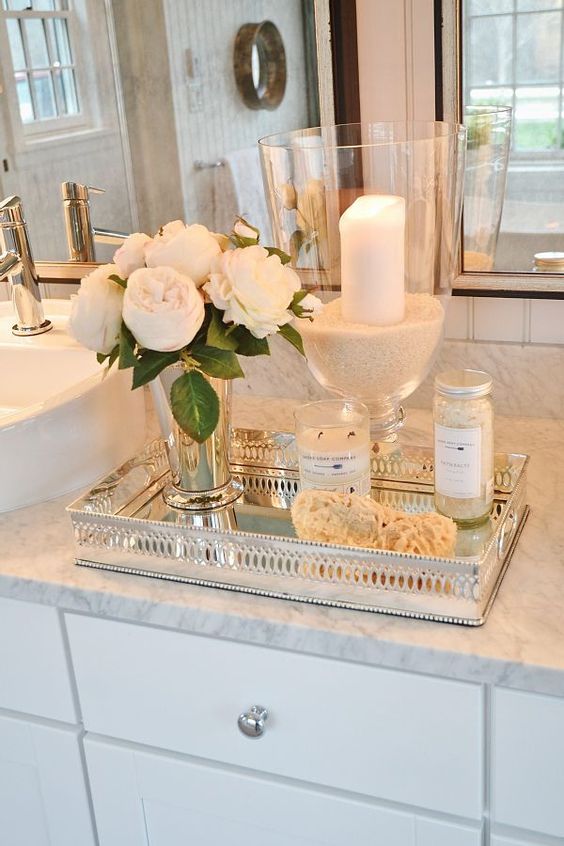This color photograph captures an elegantly designed bathroom counter crafted from white marble with intricate gray veining. Beneath the counter, a row of white drawers adorned with silver knobs can be seen. To the far left, a portion of the sink basin with a gleaming silver faucet and handle is visible. Dominating the center of the image is a sophisticated mirrored silver tray showcasing an array of decorative and functional items. 

A prominent silver vase is filled with a bouquet of exquisite white roses, their vibrant green leaves adding a touch of natural color. Adjacent to the vase stands a tall glass container, its base filled with brilliant white sand, anchoring a towering white pillar candle. The candle is lit, its wax subtly melting along the left side, casting a gentle glow. At its base sits a smaller two-wick candle encased in glass, adding further ambiance.

The tray also holds a beige sea sponge and a glass jar presumed to contain bath salts, capped with a shiny silver lid. The backdrop of this arrangement includes a large mirror reflecting the detail of a door with an inset window. On the mirrored wall hangs a stylish circular mirror, complemented by a sleek silver towel rack adorned with neatly folded white towels. This image paints a picture of luxurious and serene bathroom elegance.